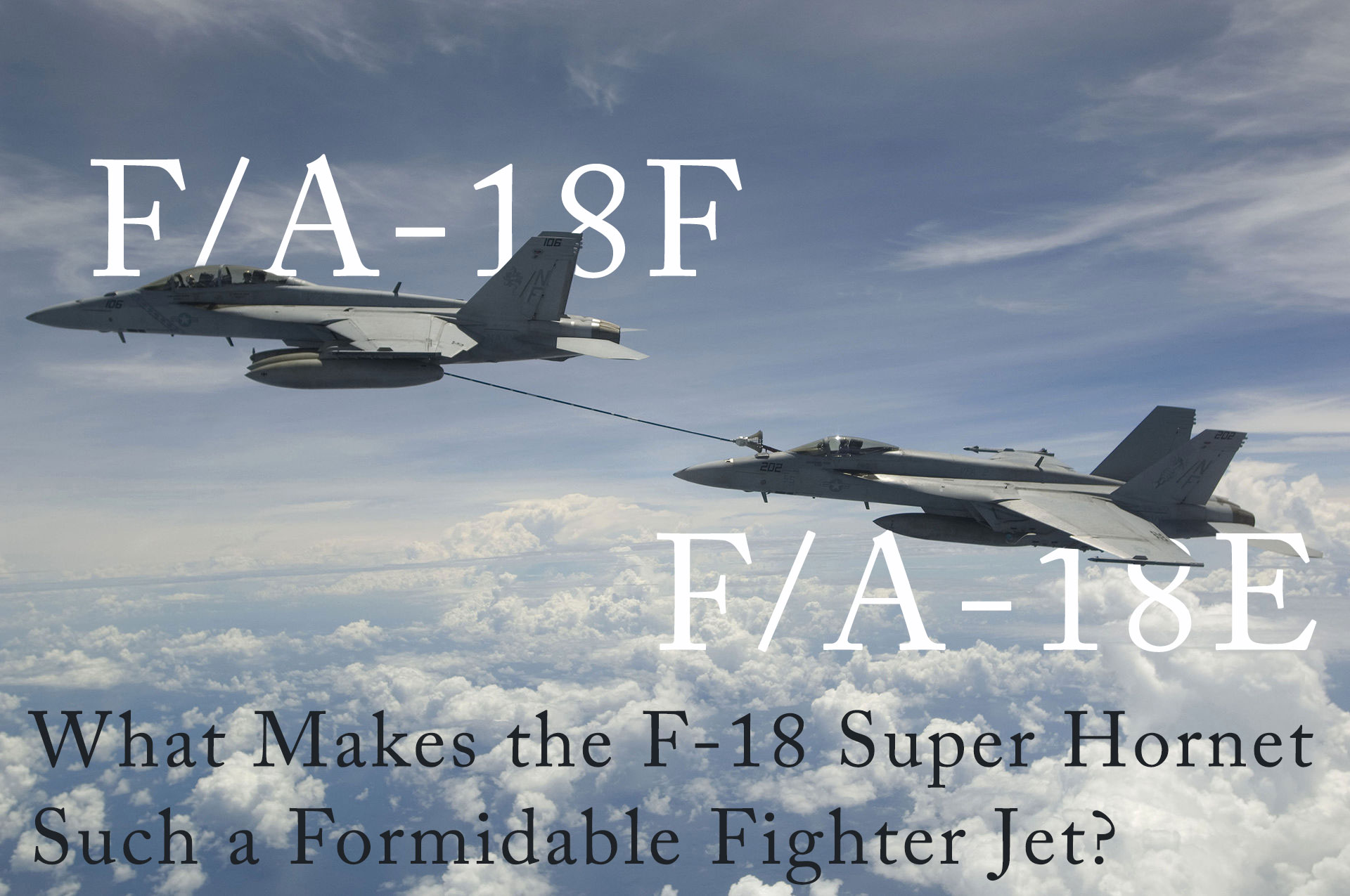The image depicts a high-altitude scene of two F-18 Super Hornet fighter jets flying in close formation in a clear blue sky surrounded by wispy and fluffy clouds. The jet on the upper left, labeled F-A-18F, is refueling the trailing jet on the lower right, labeled F-A-18E, through a black refueling line connecting the two. Both aircraft are matte gray with distinct glass cockpit domes and feature two vertical and two horizontal tail wings. The background showcases a bright sunny day with extensive cloud coverage beneath the jets. Centered at the bottom of the image, in bold black text, is the caption: "What makes the F-18 Super Hornet such a formidable fighter jet?" This graphic appears designed for informative or educational purposes, possibly for a military audience to highlight the capabilities of the F-18 Super Hornet.